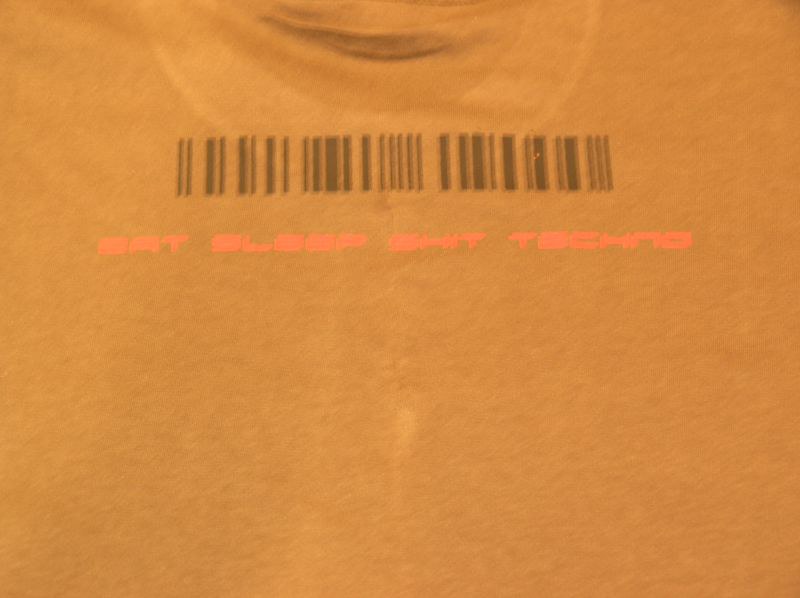This image is a somewhat blurry, close-up photograph of the front of a honey brown or gold-colored t-shirt set against an orange background. The t-shirt’s neckline appears slightly wrinkled and stretched, indicating it might be well-worn. Below the neckline, there's a black barcode that stretches across the middle of the shirt. Beneath the barcode, there is a peachy pink text that reads "Eat, Sleep, Shit, Techno." Additionally, there is a lighter, horseshoe-shaped discolored area on the fabric that could be a stain or bleach spot. The overall scene suggests a casual, possibly vintage or distressed look, and it focuses on the graphic and text design on the t-shirt.